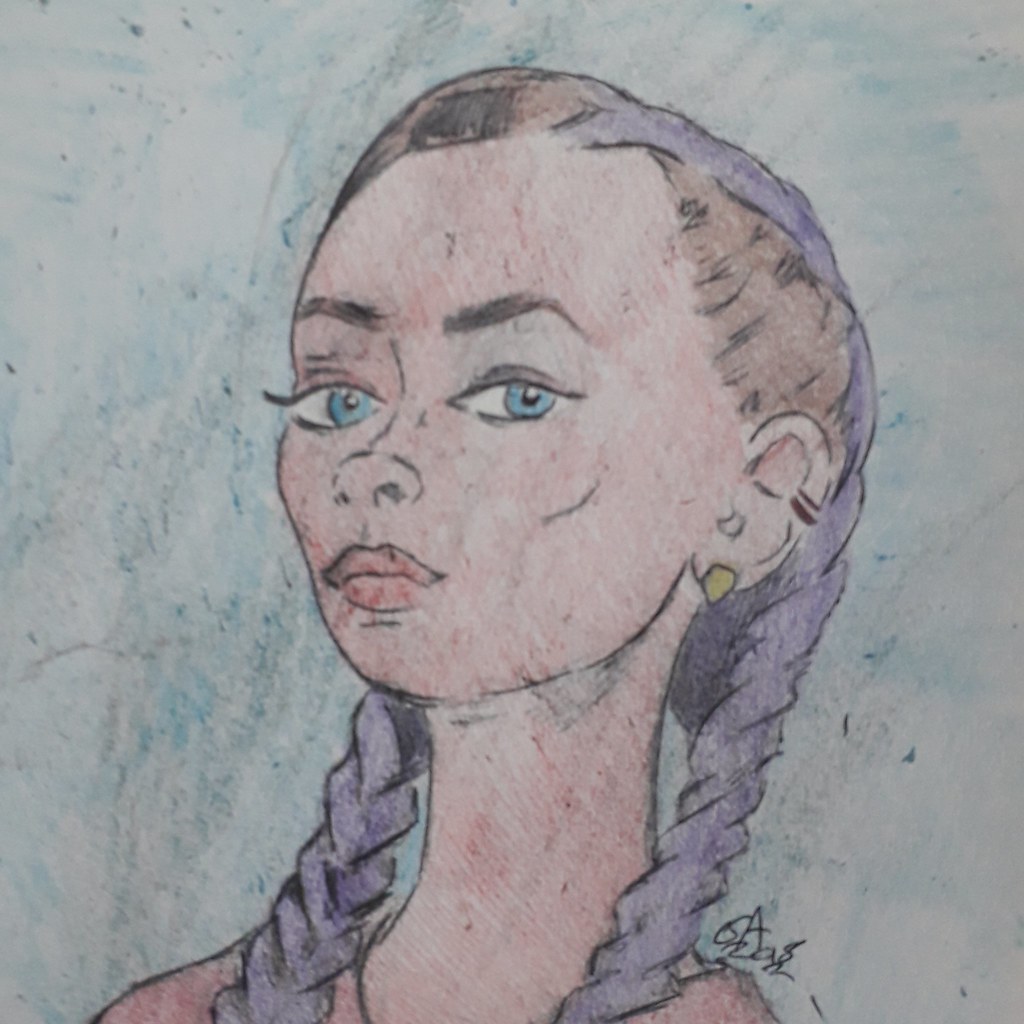This captivating artwork, rendered on a white canvas, is a striking portrait of a woman. The artist employs an intricate mix of blues, ranging from light to dark shades, interspersed with rich indigos, creating a unique and vivid background that enhances the composition's visual appeal. Central to the image is the woman's face, her piercing blue eyes seemingly locking gazes with the viewer, evoking a sense of direct connection.

Her delicate features are highlighted by a light complexion and bold, red lips, suggestive of lipstick. She wears elegant, gold diamond earrings that add a touch of sophistication to her look. Her eyebrows are meticulously shaped, hinting at recent grooming. The woman's hair is dark blonde, bordering on a light brunette, intricately styled into braided pigtails dyed in shades of purple and indigo, adding an imaginative twist to her appearance.

Despite the vivid colors and meticulous details, her expression is notably blank, creating a juxtaposition that enhances the image's enigmatic allure. Her gaze and expression combined convey a subtle, yet powerful presence that captivates and intrigues.